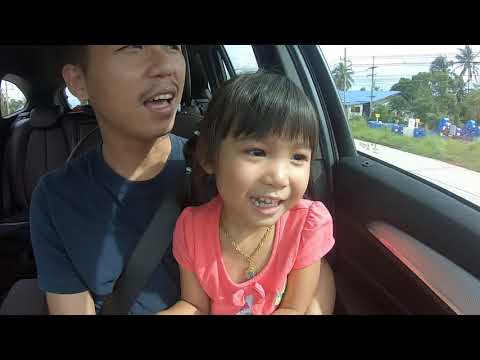The image captures a joyful moment inside a car with two passengers: a man and a young girl, who seems to be his daughter. The child is prominently centered, smiling brightly, and wearing a pink t-shirt adorned with a gold necklace featuring a pendant. She has short hair styled into bangs. The girl is sitting on the man’s lap, who appears to be a young Asian male with a slight mustache. He's dressed in a dark blue shirt and secured with a seatbelt, while the girl is not wearing one.

They are both looking out the car's side window. The car's interior is black with white trim, suggesting more seating behind the man. It's sunny outside, and the backdrop reveals palm trees, overhead power lines, and structures with a combination of blue and dark gray elements—including what seems to be a house. The presence of these elements and the vegetation gives the scene a serene, yet lively atmosphere, indicating they might be driving through a neighborhood with tropical characteristics. Both appear to be enjoying their time together, sharing a moment of happiness on their drive.